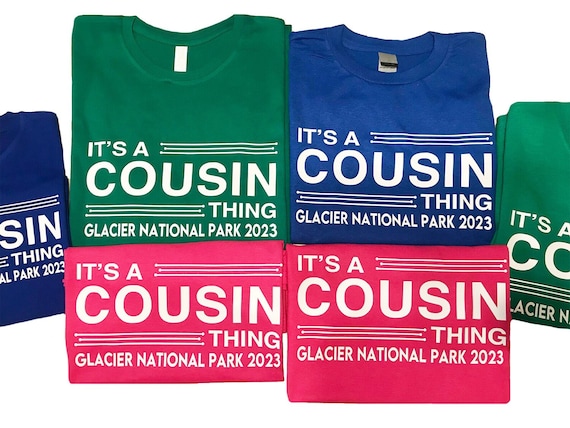This image features six neatly folded t-shirts of different colors — two green, two blue, and two reddish-pink. Arranged in two rows, four shirts are centered in the image while two are partially cut off on the edges. All t-shirts share the same design: the phrase "It's a Cousin Thing" appears prominently, with "It's a" and "Thing" in smaller letters surrounding the large, bold "Cousin" in the middle. Below this, "Glacier National Park 2023" is printed in small caps. The backdrop is a plain white, and the tags are visible on the top two t-shirts while the bottom ones are partially folded under. This composition suggests that these shirts might be custom-made for a family trip or advertised as merchandise, perhaps on a site like Etsy.